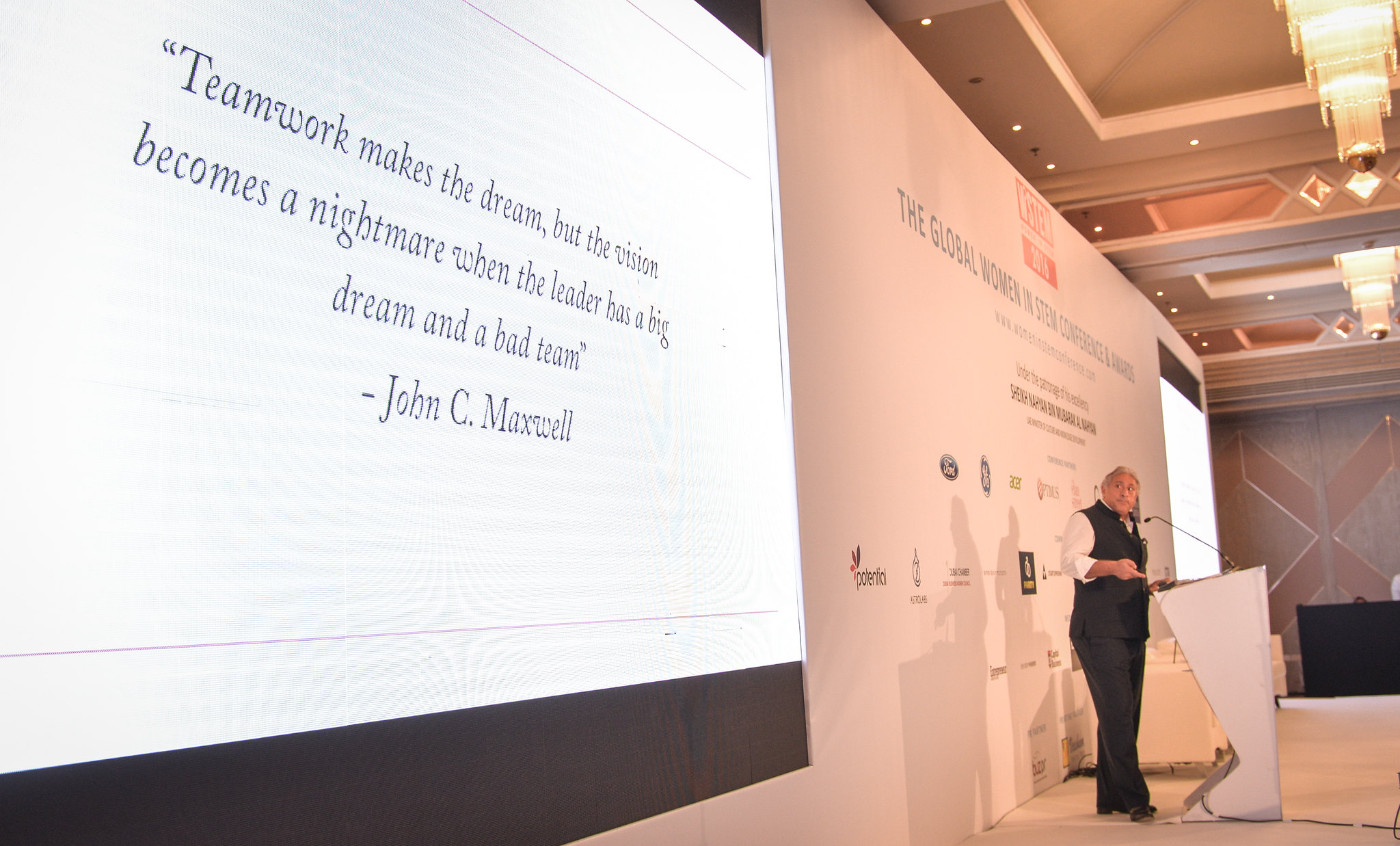The photograph captures a man giving a presentation at a lectern, dressed in a black vest, black pants, and a long-sleeved white shirt with rolled-up sleeves. Prominently displayed in the foreground is a large digital screen angled to the left, featuring the quote: "Teamwork makes the dream, but the vision becomes a nightmare when the leader has a big dream and a bad team." - John C. Maxwell. To the right of the screen, the man stands in front of a white podium, speaking into a microphone. Behind him is a backdrop with partially visible text, likely indicating the event as the Global Women in STEM Conference, accompanied by logos and a list of sponsors. The environment has a modern aesthetic with beige, gray, and brown tones, accentuated by sculptural chandeliers hanging from the ceiling. The overall scene exudes a monochromatic feel with deliberate splashes of color, emphasizing the importance of promoting women in STEM fields.